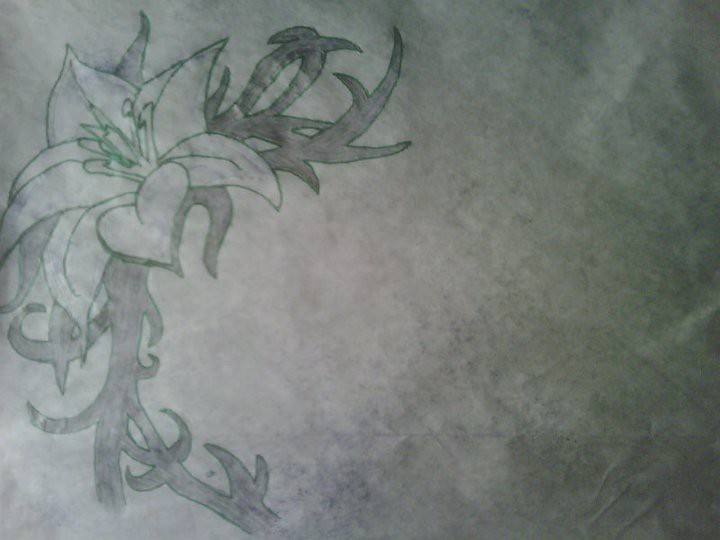The image depicts a piece of special drawing paper, around 30% wider than it is tall, with noticeable diagonal wrinkles and dirt marks concentrated in the bottom right corner, casting various shadows across the off-white background. Dominating the left side of the image, a detailed sketch of a flower catches the eye. The flower, featuring six petals, is outlined in green and boasts intricate pollinator details at its center. Surrounding the flower is a mix of greenery shaded in purple and long, thorny branches. The overall composition suggests an attempt at designing a tattoo, with the artwork slightly off-center and the paper’s texture contributing to a realistic, tactile feel.